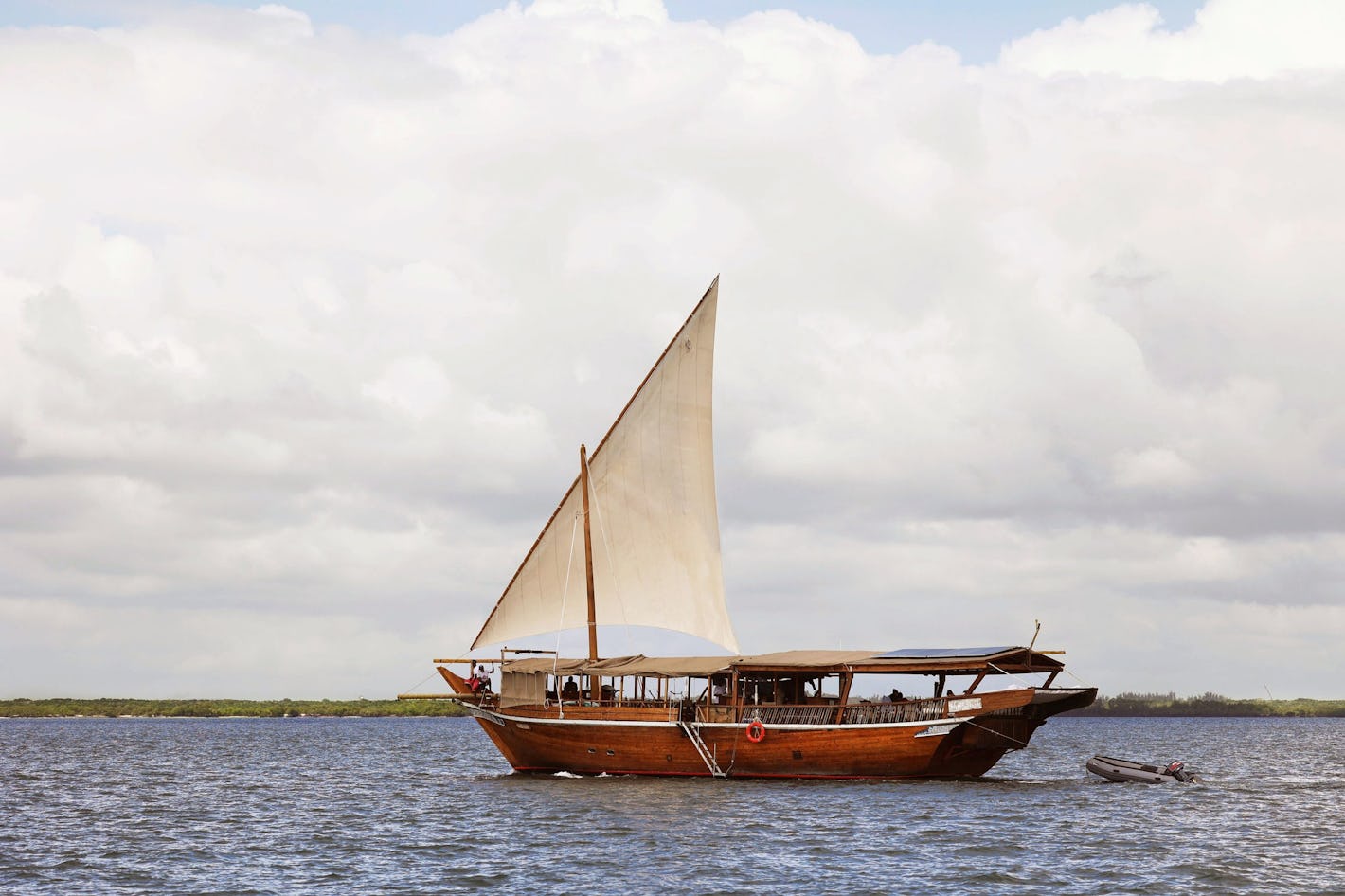The photograph depicts a red sailboat navigating a large body of water, potentially a lake or bay. The sailboat has a white sail prominently positioned in the center of the image, resembling a right triangle against a backdrop of the horizon. The boat also has a low roof structure, and its wooden hull hints at traditional craftsmanship. Behind the sailboat, to the right side of the image, a smaller gray inflatable raft is being towed, though it is unclear if it is connected by a rope. There are people visible inside the boat near the anchor, and an orange life float or tube is hanging on its side. The water, dark grey in color, occupies about 20-25% of the lower part of the image, while the majority of the upper part is dominated by a blue sky filled with dense, fluffy white clouds. In the distance, a green shoreline can be seen, adding to the serene and picturesque sailing scene.